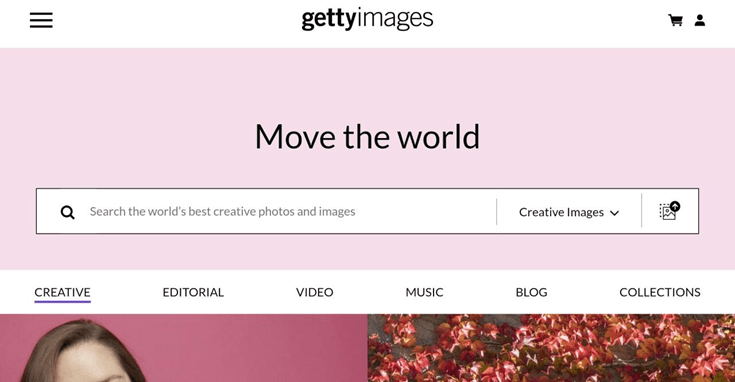In this image, the layout includes various UI elements and details, enhancing its functionality and aesthetic appeal. At the very top, there are some blurred or unclear images. On the top-right corner, there is a cart icon, indicating a shopping feature, while the top-left corner has a menu button for navigation. Just below these elements, the text "Move the World" is prominently displayed, providing an inspirational touch.

Centrally positioned is a search field inviting users to "Search the world's best creative photos and images" which emphasizes the platform's extensive collection. Below the search bar, there are clearly marked categories including Creative, Editorial, Video, Music, Blog, Collections, each designed to streamline user experience and exploration.

The image features a vibrant pink color scheme, adding a lively and engaging visual. Notably, at the bottom left, there's a half-visible human face, likely of a woman, which adds a personal and intriguing element to the overall design. The meticulous arrangement and color choice contribute to an inviting and user-friendly interface.